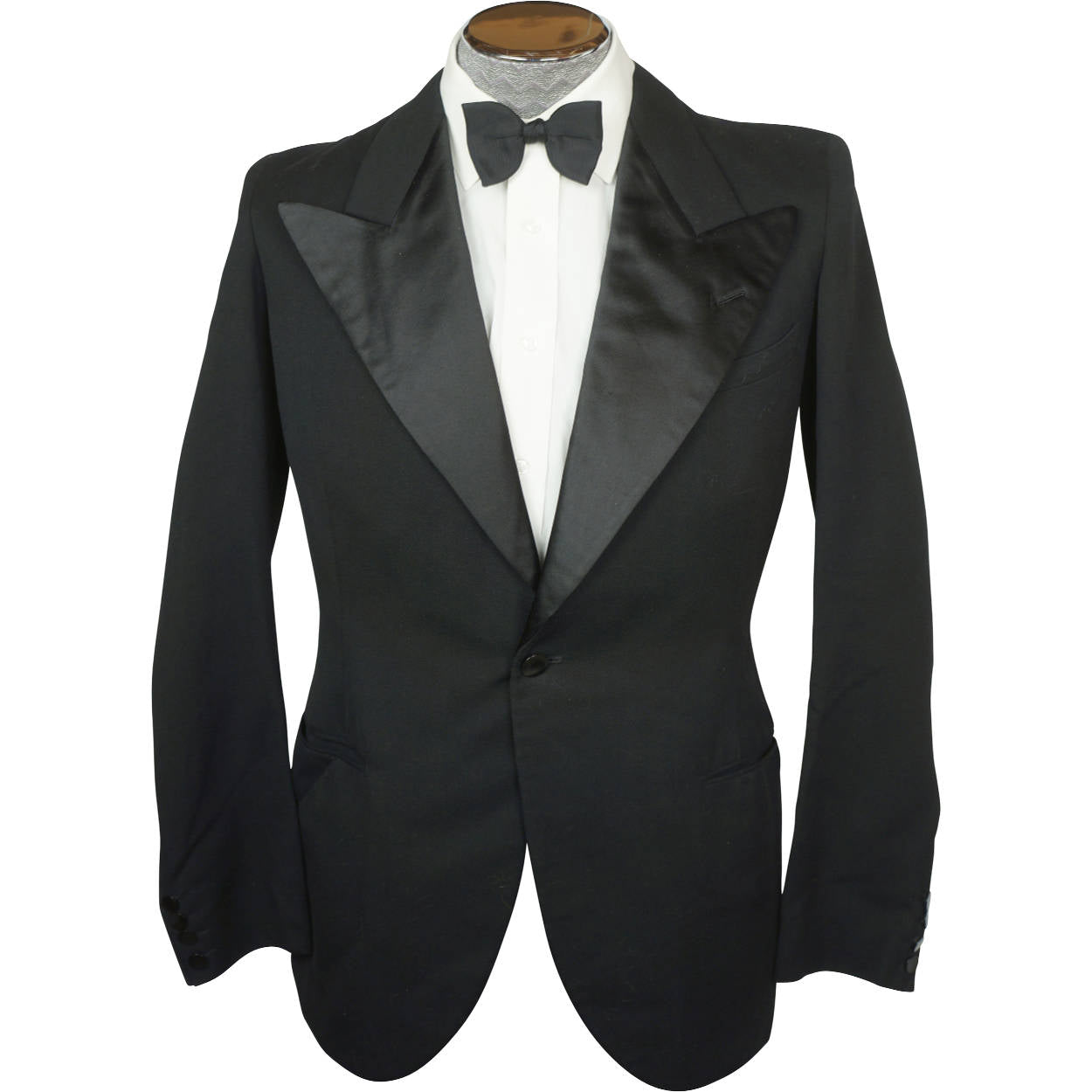The image features a sophisticated tuxedo ensemble displayed on a headless mannequin. The tailored tuxedo jacket, crafted from matte black fabric, boasts wide lapels adorned with luxurious black satin. A single button secures the jacket at the waist, enhancing its sleek, streamlined appearance. Underneath, a pristinely pressed white dress shirt is meticulously showcased, highlighting its broad front placket and neatly starched collar. A classic black bow tie, perfectly fastened at the mannequin's neck, completes the formal look. The mannequin itself, made from a material that appears either grey or pale silver, sports a distinctly brown neck opening, accentuating the contrast of the ensemble's elegant details.